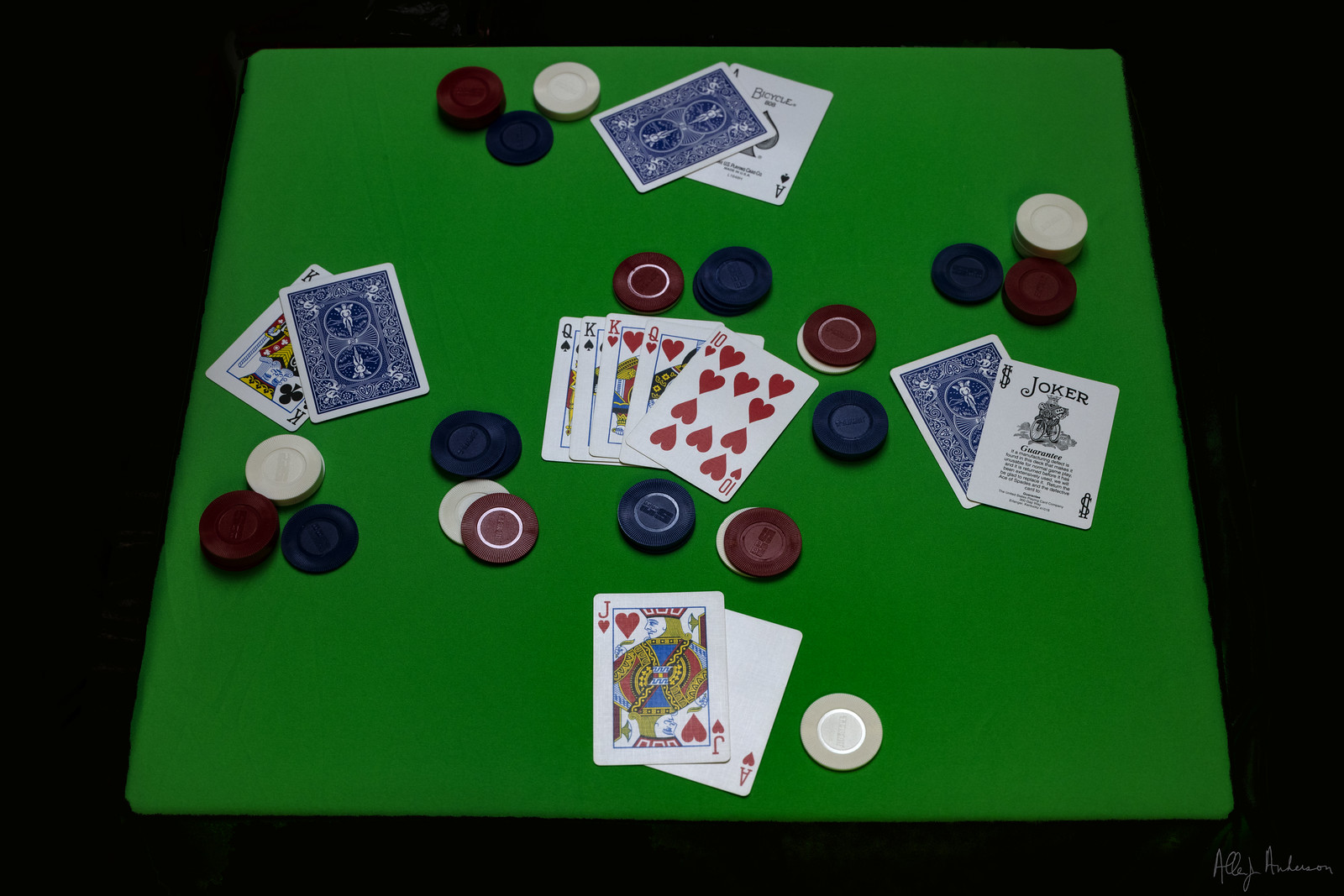This 3D rendered image captures a tense poker game scene from a bird's-eye view. The square, green felt poker table is central to the composition, surrounded by a stark black background that emphasizes the focus on the game. At the center of the table, five community cards lie face-up, displaying a queen, two kings, another queen, and a ten, indicating a potentially high-stakes hand.

Each side of the table represents a player’s position, though no players are physically present. Various red, blue, and white poker chips are scattered around the table, adding to the tension of the moment. 

Each player has been dealt two cards. The bottom player’s cards are fully visible, revealing a jack and an ace, suggesting a strong hand. In contrast, the other three players have only one card face-up each: the left player shows a king, the right player reveals a joker, and the top player displays an ace. Their second cards remain face-down, adding an air of mystery and anticipation.

Along the bottom right corner of the image, the artist's signature is present, though it is too fine to be legible from this angle. The rendering is so meticulous that it blurs the line between digital creation and reality, with the only discernible shadows cast by the poker chips, adding depth and dimension to the scene. This intricate depiction invites viewers to immerse themselves in the intensity of the moment, pondering the possible outcomes of the game.